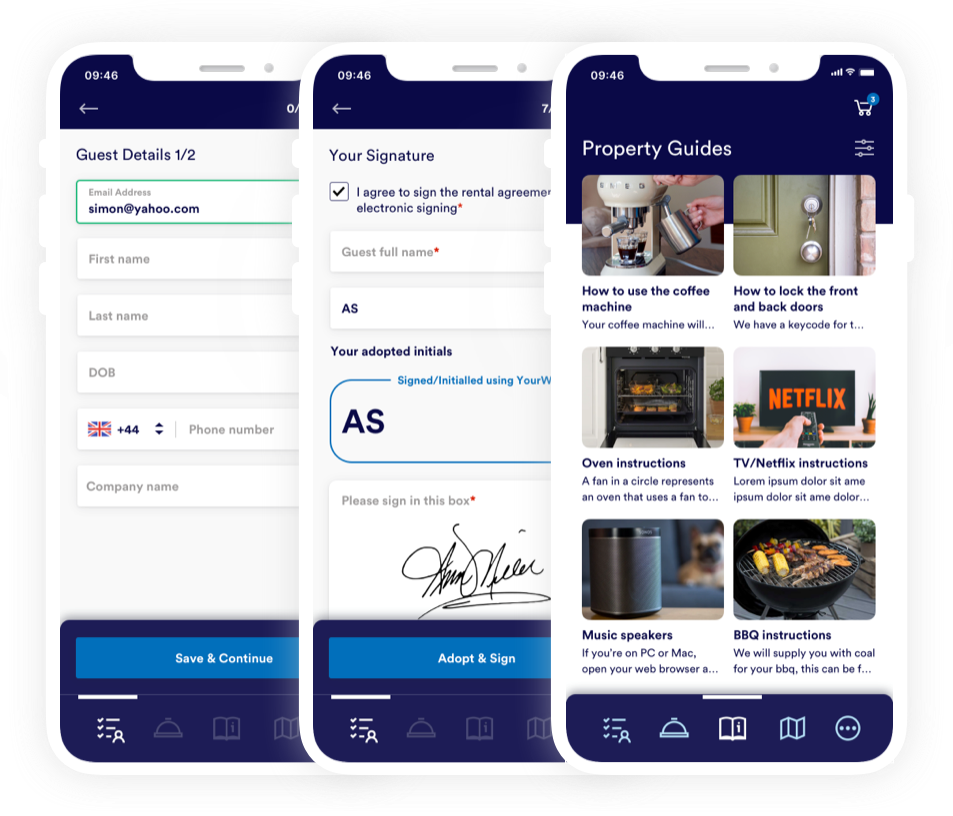### Detailed Caption:

This image features a series of three simulated cell phones, each with distinct screens and details, but unified by a consistent design theme. Each phone is white with a white notch at the top. 

1. **First Cell Phone Screen**:
   - **Top Section:**
     - The time on display is "9:46".
     - Includes a white back arrow on the left.
     - A navy banner is present with white text.
   - **Main Content:**
     - A white background with navy font and a section titled "Guest Details 1 of 2".
     - Below the title, there's a green-highlighted box with the email "simon@yahoo.com".
     - Several white input boxes are labeled for "First Name", "Last Name", and "DOB (Date of Birth)".
     - Displays the British flag (Union Jack) next to a phone number box marked with "+44".
     - Options for "Company Name" are present.
   - **Bottom Section:**
     - A navy banner features a blue and white button labeled "Save and Continue".
     - Underneath are icons for a list with a person, a dinner dish, a book/newspaper, and similar icons as the other phones.

2. **Second Cell Phone Screen**:
   - **Top Section:**
     - The same navy banner and white back arrow found in the first phone are present, with the time "9:46".
   - **Main Content:**
     - Displays a signature box with a black cursive signature and the instruction "Please sign in this box."
     - Above the signature box, it reads "Sign Initial Using: AS" in blue.
     - Another section labeled "Your Adopted Initials" with a white box containing "AS" in navy.
     - Below, a gray box marked "Guest Full Name" with a red asterisk. 
     - Agreement clause stating, "I agree to sign the rental agreement electronically", with a red asterisk.
     - A white box with a blue checkmark for "Your Signature".
   - **Bottom Section:**
     - Mirrors the first phone's navy banner but with the text "Adopt and Sign".
     - Contains the same series of icons as described earlier.

3. **Third Cell Phone Screen**:
   - **Top Section:**
     - The same time "9:46" is displayed, along with a Wi-Fi icon and a battery indicator.
     - Displays a white cart icon with a blue "3".
     - Reads "Property Guides" in white, followed by various lines and images.
   - **Main Content:**
     - Series of images provide instructions:
       - "How to use the coffee machine" with an image of a hand using the machine.
       - "How to lock the front and back doors" showing a key in an olive door.
       - "Oven Instructions" displaying a fan icon within a circle and a black oven with food inside.
       - "TV Netflix Instructions" with a person's hand holding a remote and a Netflix screen on a TV.
       - "Music Speakers" showing a black cylinder, with instructions for PC and Mac users.
       - "Barbecue Instructions" accompanied by a picture of corn and meat on a grill.
   - **Bottom Section:**
     - The navy bar with the same icons as previously mentioned.

Each phone's screen provides a different form of interaction, from filling in guest details to signing documents, and offering property guides with visual instructions, all unified by consistent design elements.